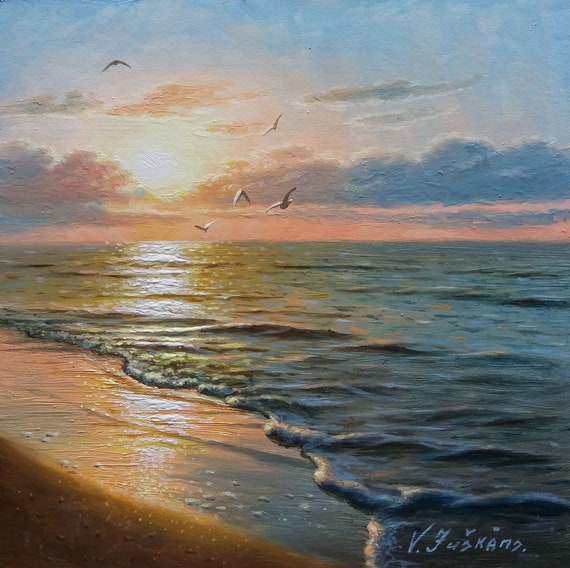The painting is a vivid and realistic seascape on a square canvas, capturing a serene beach at dusk. The ocean rolls gently onto the golden brown sand, its waves breaking softly and creating subtle indentations and water bubbles as they reach the shore. The sky is a mesmerizing blend of orange, peach, and blue hues, with the setting sun casting its radiant light and reflecting on both the sand and the water. The clouds, colored in pinkish-blue and orangish tones, stretch horizontally across the sky. In the distance, five seagulls can be seen flying towards the sun, adding a touch of life to the tranquil scene. The painting is signed in the lower right corner with a light blue font, presumably by an artist whose name appears to begin with a "V" and might say "B. Pushkant." The exquisite details and harmonious colors accentuate the beauty of this captivating seascape.